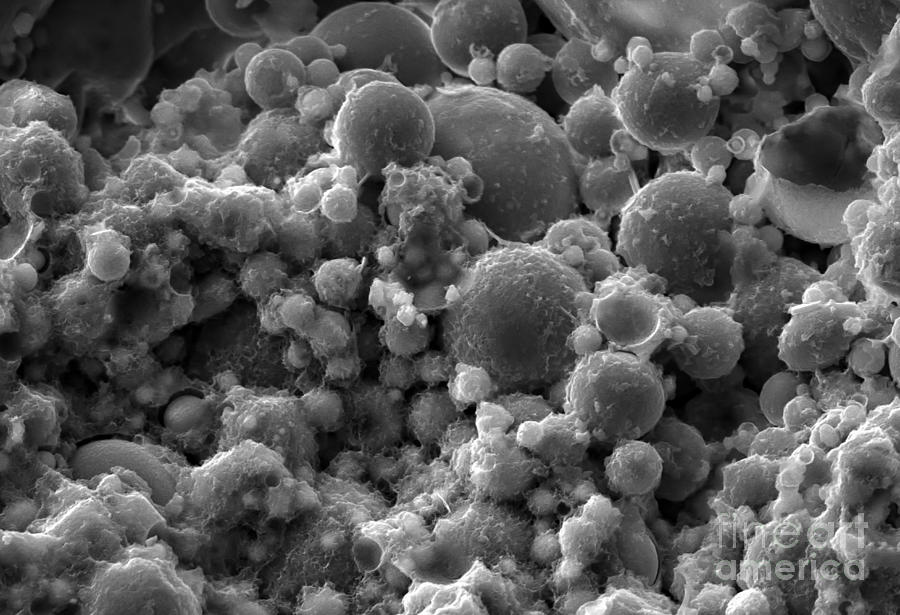The image is a highly magnified black and white photograph, likely taken through a microscope, featuring a multitude of spherical objects varying in size from very tiny, comparable to grains of couscous, to larger ones about the size of peas. These spheres are predominantly clustered together, adhered by a sticky substance, possibly resembling eggs embedded in an embryonic fluid. The photograph contains a mix of light and dark gray spheres, with light reflections visible on some of them, particularly in the bottom half. A notable area in the upper left-hand corner has a darker background compared to the rest of the image. In the bottom right corner, the watermark "Fine Art America" appears in ghosted white font.